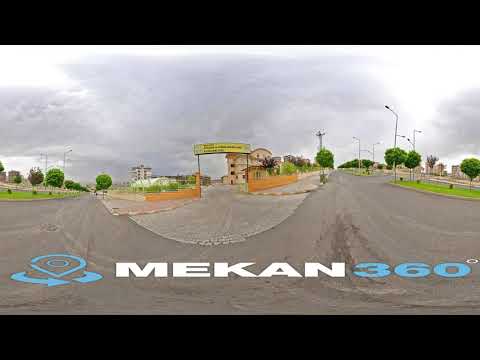The photograph, taken outdoors in the middle of the day, showcases a wide street scene under a cloudy sky. At the top and bottom of the image are solid black horizontal bands. In the center of the image, a roadway stretches forward with a light gray walking space down the middle, surmounted by a yellow banner with indistinguishable black text. The surrounding area features various buildings, grassy sections, and distinctive lollipop-shaped trees in the background. At the bottom of the photograph, superimposed text in white and blue reads "MECAN 360 degrees," with "M-E-C-A-N" prominently capitalized. The overall colors of the image include black, white, gray, yellow, orange, green, and light blue, captured in a fisheye view that creates a slightly curved effect. The scene is notably devoid of people and vehicles, giving it an almost serene, empty ambiance.